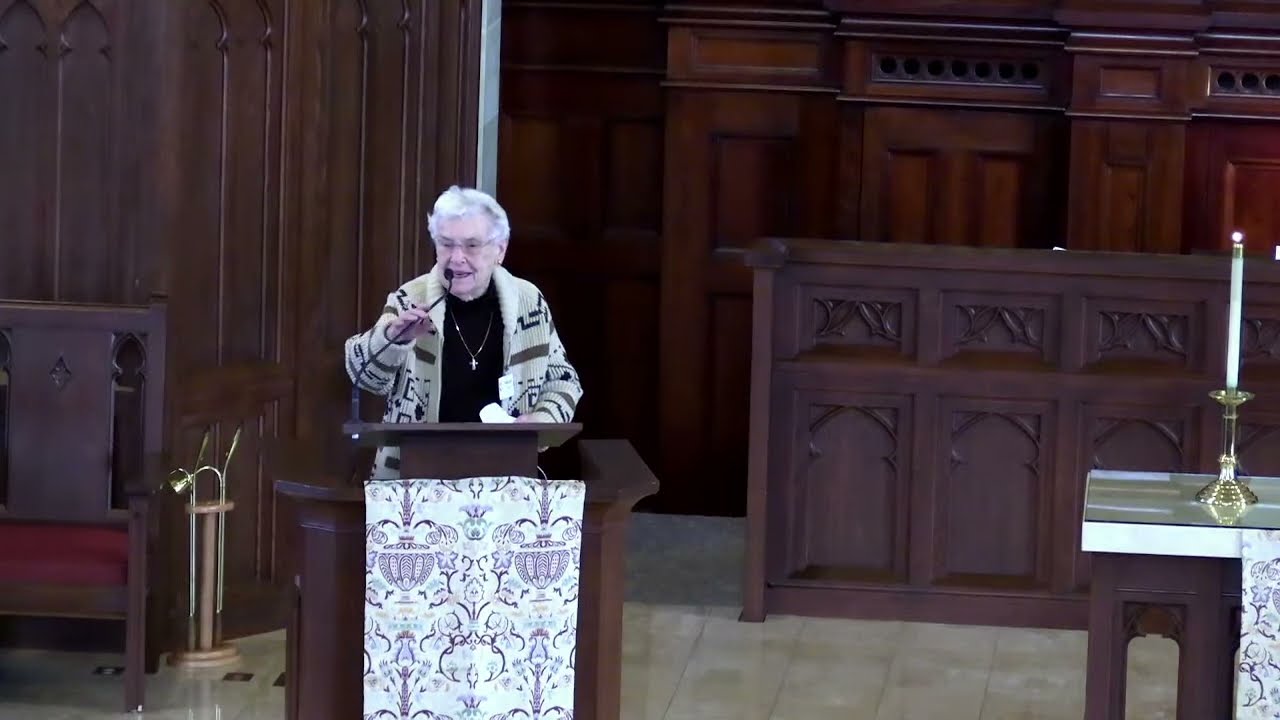Inside a church with rich, dark wooden furniture and walls, an old woman stands at a wooden podium adorned with a white fabric banner bearing black drawings and symbols that hint at a religious theme. She has short white hair and wears glasses, a black shirt with a gold cross necklace, and a jacket that is mostly white with indiscernible black designs. Her left hand holds a piece of paper on the podium while her right hand holds a microphone attached to it, positioned directly in front of her face. The floor beneath her is a polished stone, and to the far right, a table with golden candlestick holders and lit candles can be seen, adding to the church's sacred ambiance.